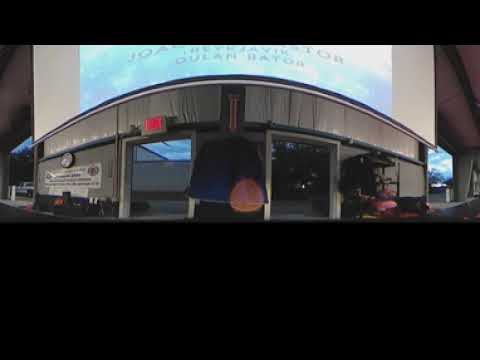The image depicts a panoramic shot of a building that appears to be situated on a street corner, giving the impression of both an indoor and outdoor exhibit thanks to some fisheye-style distortion. The structure, which resembles a storefront or possibly an industrial loading dock, has two large entryways devoid of doors, allowing a clear view inside. The interior features concrete floors and walls, with the upper portion painted in a maroonish-brownish hue. A clock and a white banner adorn the wall to the left, while some clutter, including pink and black items, can be seen on the right. There is also a large garage-style door on the right side of the building. 

Dominating the scene is a very large screen positioned above the structure, projecting an unclear image that might be an elaborate sign or related to a drive-in theater. The lack of visible sidewalks or streets around the building, coupled with the dark exterior, gives the impression of the building floating in an ambiguous space. The overall scene, blending indoor and outdoor elements at dusk, suggests that this could be an attraction of some sort, possibly within a larger industrial or exhibit area.